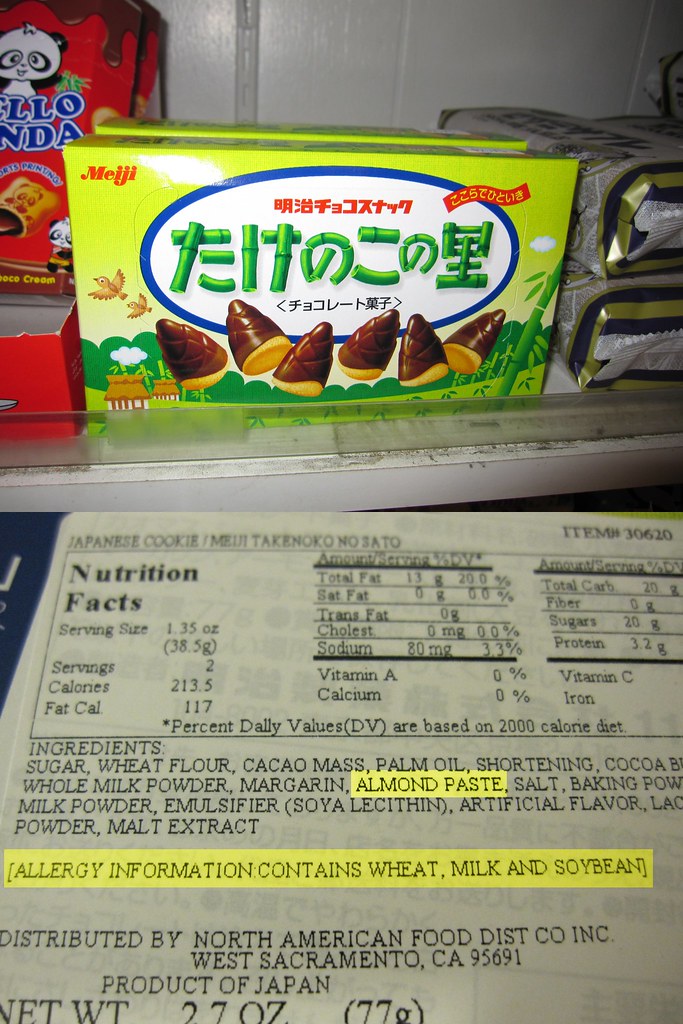This color photograph showcases a variety of Japanese snack items displayed on a shelf. Central to the image is a green box adorned with Japanese writing and featuring an array of cone-shaped chocolates. The box prominently displays the word "Meiji" in the top left corner. The chocolates, appearing to have slimy caramel bits poking out, are reminiscent of small snail shells or eggs. Situated to the left of the green box is a red package of Hello Panda cookies, easily identifiable by the cartoon panda above the brand name. Below the green box, a detailed nutritional label provides specifics: serving size 1.35 ounces (38.5 grams), with 2 servings per box, totaling 213.5 calories each, 117 of which are from fats. The ingredients listed include sugar, wheat flour, cacao mass, palm oil, shortening, whole milk powder, margarine, and almond paste, the latter being highlighted in yellow. Also highlighted is the allergy information, indicating the presence of wheat, milk, and soybeans. This product is distributed by North American Food Distribution Company, Inc., West Sacramento, California, 95691 and has a net weight of 2.7 ounces (77 grams).